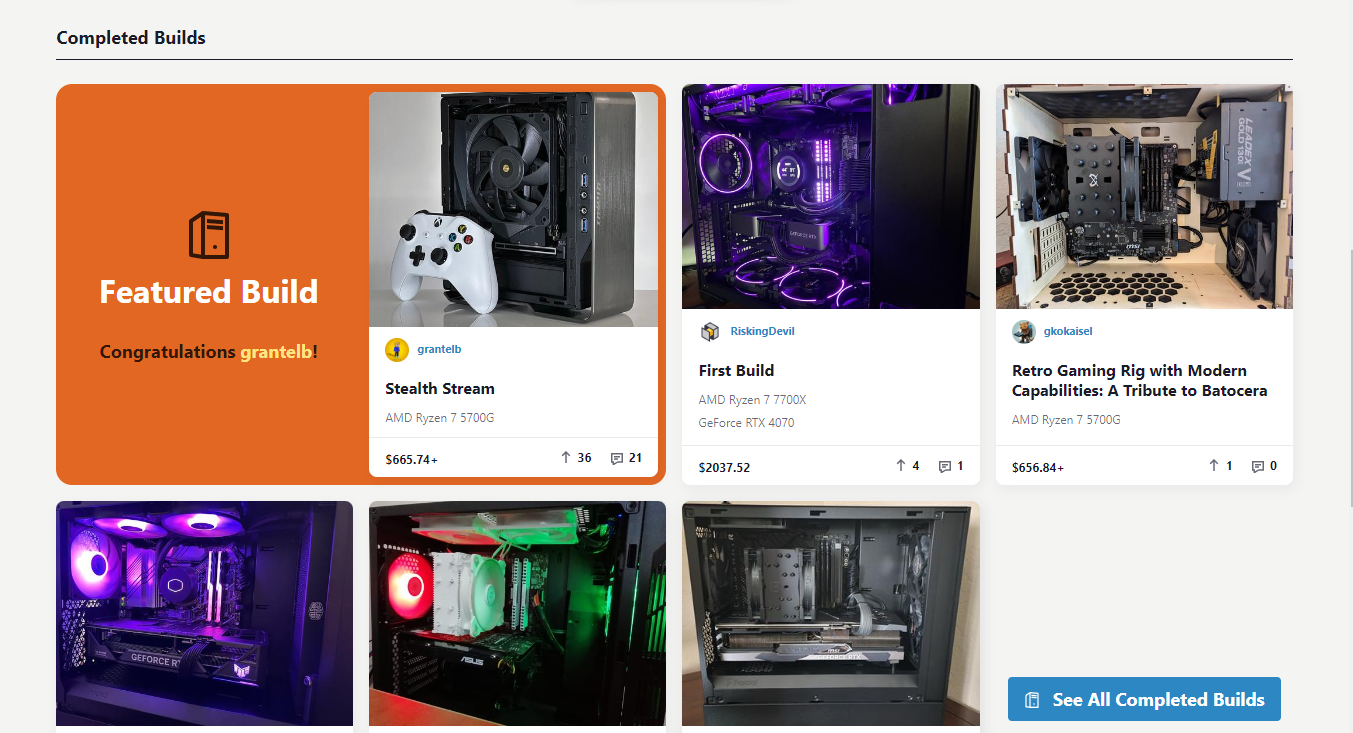The image showcases an array of completed computer builds. In the upper left corner, the title "Completed Builds" is displayed prominently in bold font, separated from the rest of the content by a thin black line. Below this, six images of completed computer builds are arranged in a grid.

On the left-hand side, highlighted in an orange box, is the "Featured Build" section. It congratulates Grant Albee on his build, titled "Stealth Stream." This particular build includes a prominent computer case with a controller resting against it. The specifications listed indicate it's powered by an AMD Ryzen 7 5000G processor, and it has received 36 upvotes and 21 comments.

Adjacent to the "Featured Build," we see a build labeled "First Build," which features an AMD Ryzen 7 7700K processor. The detailed organization and stylized presentation offer a clear and engaging overview of various high-quality computer builds.